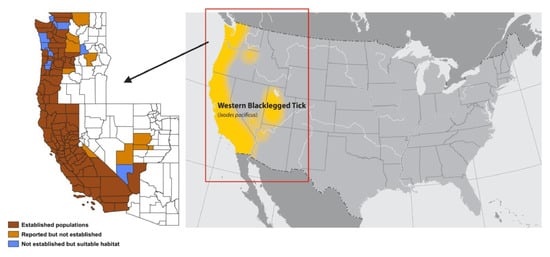The image is a detailed map illustrating the distribution of the Western Black-Legged Tick in North America. The primary map displays the United States in light grey, with Canada and Mexico in darker grey, with all water bodies in even lighter grey. The west coast, including California and parts of neighboring states like Oregon and possibly Arizona, is highlighted in yellow. Accompanying this main map, there is an enlarged inset to the left depicting California and parts of the nearby states. California is notably shaded almost entirely in dark brown, indicating regions with established tick populations, as per the map's legend. Other areas within the highlighted states vary in color: light brown for reported but not established locations and blue for regions that are not yet established but are considered usable habitats. The text "Western Black-Legged Tick" is prominently displayed on the west side of the primary map along with an annotation that includes a hard-to-read section beneath it. This detailed visual aid is bordered by a thin brown rectangle with an arrow pointing to the inset map, providing a clearer breakdown of the tick's habitation zones across the counties.